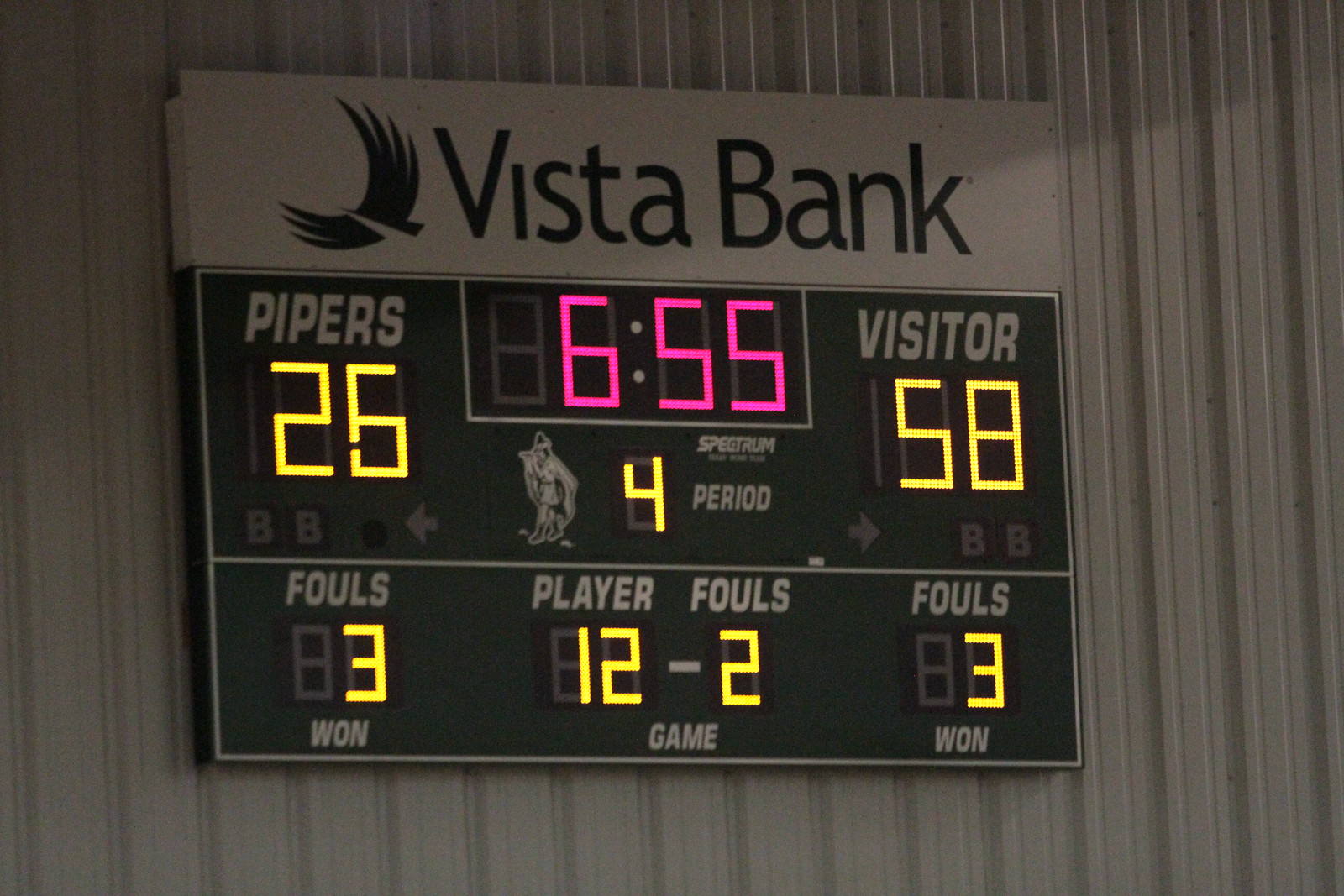The photograph captures a digital scoreboard mounted on a white corrugated steel wall. The scoreboard, predominantly green with white font, features the branding "Vista Bank" at the top in dark green text. An abstract green bird icon is situated to the left of the brand name. The scoreboard displays several game statistics: on the left side, it reads "Pipers 26" in yellow LED digits; the central section shows the time "6:55" in pink LEDs, followed by "4th period" in yellow LED text. The right side of the scoreboard indicates the visiting team's score as "Visitor 58" also in yellow LEDs. Additional game details at the bottom include "Pipers 3 Fouls, Visitor 3 Fouls, Player 12, 2 Fouls." The entire setup maintains a clean and structured appearance against the white metal backdrop.